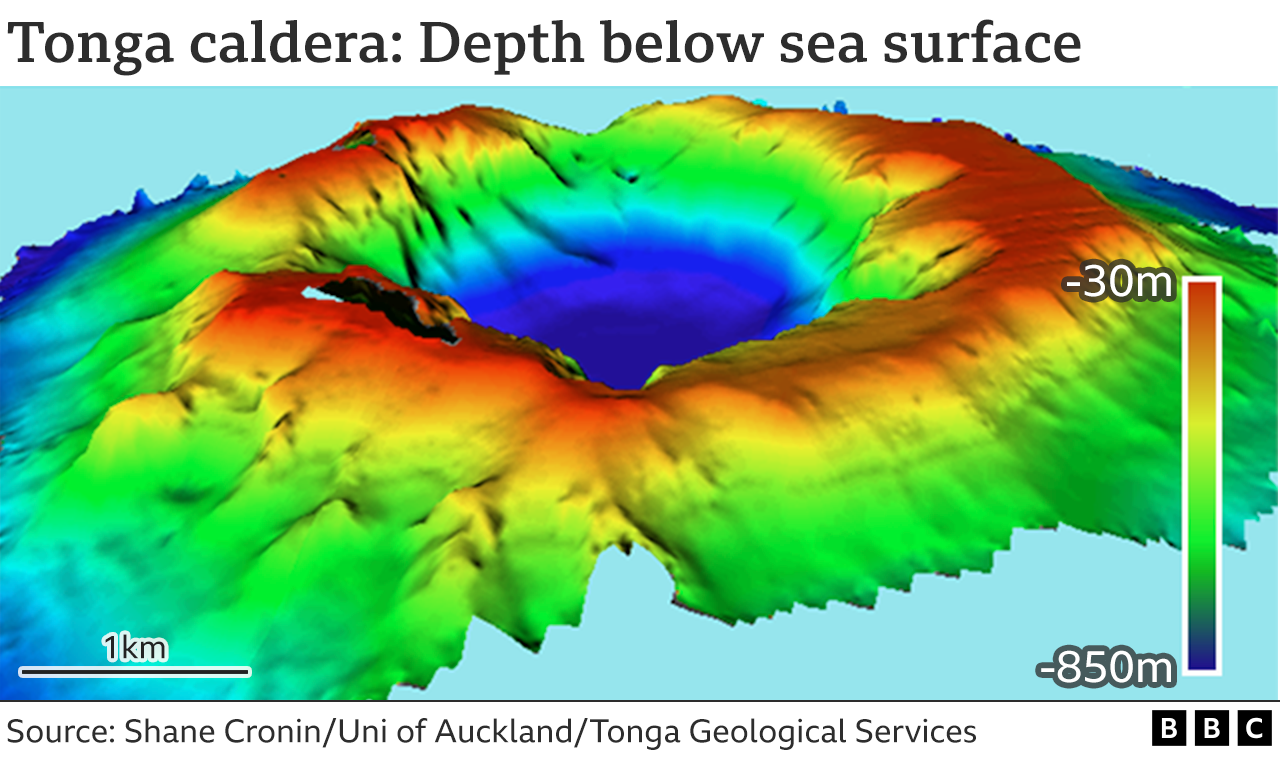This detailed infrared map, labeled "Tonga Caldera, Depth Below Sea Surface" at the top, is from the BBC, with their logo displayed in the bottom right corner. The image depicts an overhead view of a volcanic structure with a central caldera, represented in a rainbow color scheme akin to a heat map. The depth map, set against a blue background with a white border, illustrates varying depths signified by different colors, ranging from red at shallower depths (-30 meters) to blue at greater depths (-850 meters). The caldera itself features a bowl-shaped depression with dark blue indicating the deepest sections. Surrounding this, the depth transitions through green towards the center, and reds and oranges are prominent along the upper rim. Moving outward, the colors shift back through yellows and greens to blues again, indicating shallower depths at the structure's base. A depth key on the right side of the image provides a reference for interpreting these color gradations. Additionally, on the white background beneath the map, credit is given to Shane Cronin, the University of Auckland, and Tonga Geological Services. A scale representation indicating one kilometer is also included at the bottom left.